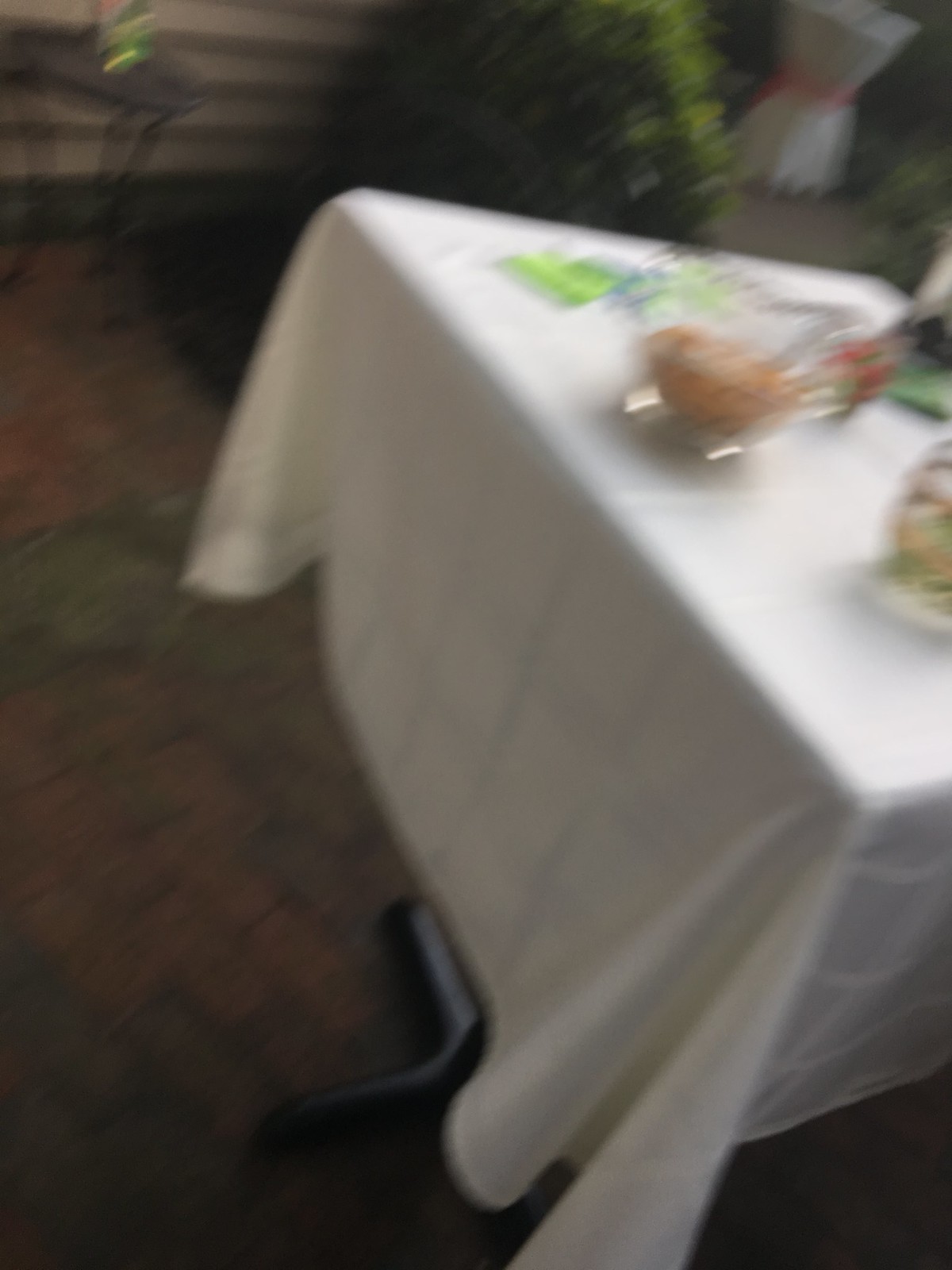This color photograph captures a small serving table dressed in a crisp white tablecloth. Various items, including folded napkins, are spread across the tabletop, though the specific dishes are indistinct. A small, peachy-orange serving bowl draws attention with a set of spoons protruding from it. The table stands on a pedestal base, which rests upon a floor with a brick-like appearance, suggesting an outdoor setting. In the upper left of the frame, a piece of wrought iron furniture can be seen, while greenery decorates the top right, contributing to the ambiance. The image seems to depict either a table in the process of being set up or one that has been recently vacated, as suggested by the scattered objects and possible menus. The overall scene is blurred, making fine details difficult to discern.